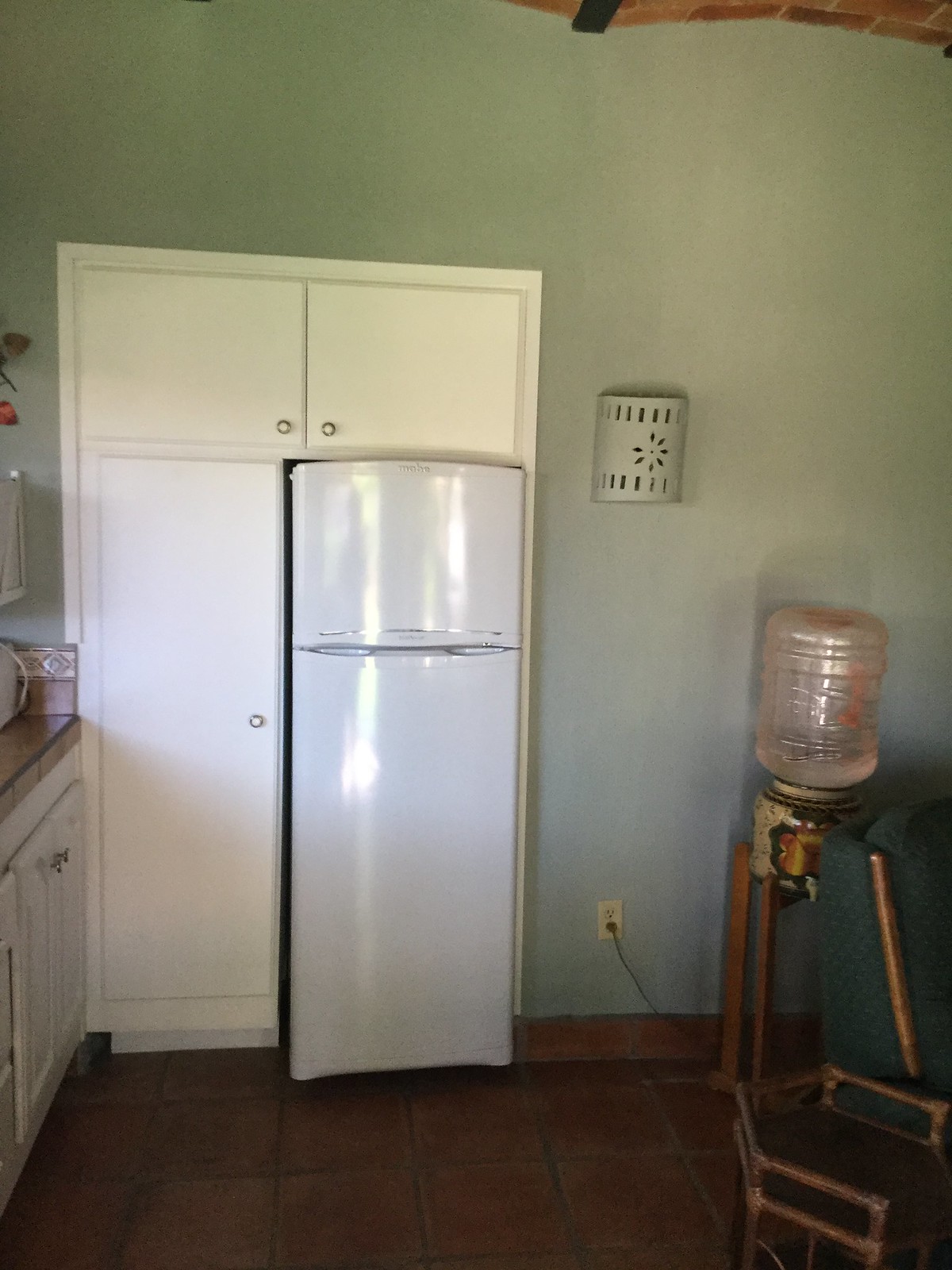The image depicts a section of a kitchen with a distinct retro charm. The walls are painted in a light green hue, providing a soft backdrop for the scene. Prominently featured is a compact yet bulky white retro-style refrigerator, neatly fitted into its designated space. Surrounding the fridge are multiple white cabinet doors, including two atop the refrigerator and a long cupboard alongside it. To the left of this setup, a beige countertop is partially visible, with two cabinets situated beneath it. Adjacent to the fridge is an older-style water cooler, characterized by its clear container and brown base where water is dispensed. Additionally, the kitchen accommodates a small wooden coffee table and a chair with a green cloth, possibly denoting a dining nook. Above this area, a wall sconce provides lighting, while an outlet near the tiled floor has something plugged into it. The scene is completed with the sight of what seems to be a sink area next to the refrigerator, further framed by more cabinets.